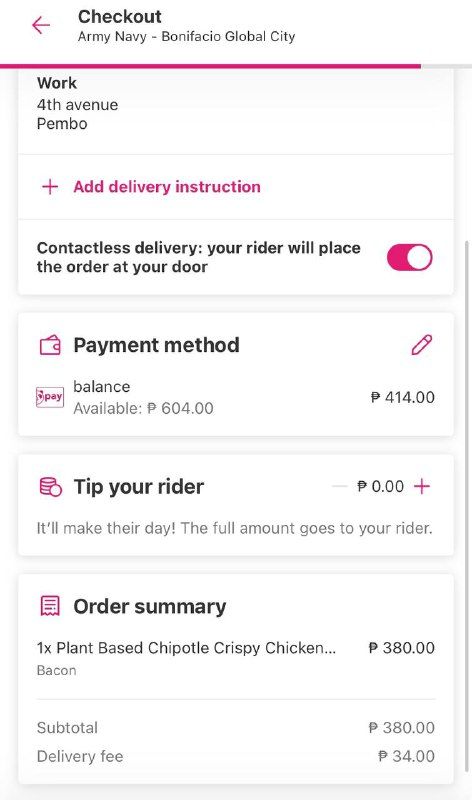**Caption:** 

The screenshot features a user interface on a white background, likely from a food delivery app. Prominent on the screen is a "Check Out" button highlighted with a leftward arrow. A list of locations — Army, Navy, Winnebago, Global City, BONIFACIO, Spork, 4th Avenue, and Pembo — appears, suggesting delivery options or possible addresses.

Below, there’s an option to "Add Delivery Instructions" with text indicating "Contactless Delivery," assuring that the rider will place the order at the door. A toggle bar (currently deactivated) is visible, denoting some form of toggleable option.

The "Payment Method" section includes an editable pencil icon, showing a balance available of ₱604. There’s also a "Tip Your Rider" section starting at ₱0.00, with increment and decrement buttons right next to it, alongside a note reassuring that the full tip amount will be given to the rider and a reminder that "it'll make their day."

At the end of the caption is the order summary, noting "1x Plant-Based Chipotle Crispy Chicken..." priced at ₱380, followed by a subtotal of ₱380 and a delivery fee of ₱34. There’s also a "Grace" progress bar to the right, likely indicating order preparation status or delivery progress.